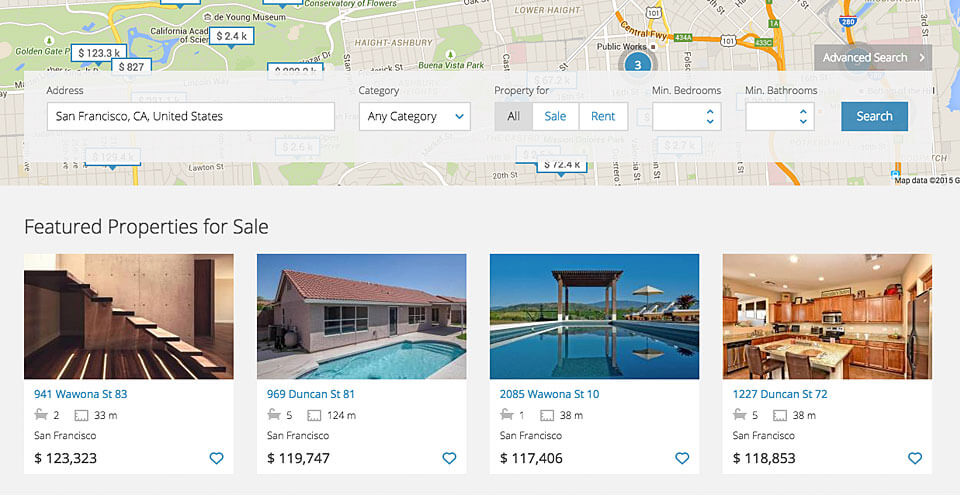A detailed caption for the given image could be:

"A screenshot of a real estate website featuring a top navigation bar and a map with green and taupe-gray backgrounds, showcasing streets, landmarks, and waterways. The interface includes a comprehensive search bar labeled 'Address,' set to 'San Francisco, CA, United States,' with a category filter (set to 'Any category') and property type option (set to 'All'). Users can select between 'For Sale' or 'Rent' in blue text, choose minimum bedrooms and bathrooms from the drop-down menus, and initiate the search with a blue button featuring white text.

Below the search bar, the website highlights 'Featured Properties' with a title, each word beginning with a capital letter. Four property images are displayed with their respective details:
1. '941 Wawona Street #83, San Francisco, $123,323.'
2. '969 Duncan Street #81, San Francisco, $119,747.'
3. '2085 Wawona Street #10, San Francisco, $117,406.'
4. '1227 Duncan Street #72, San Francisco, $118,853.'

The layout is clean and user-friendly, facilitating easy navigation and property searches."